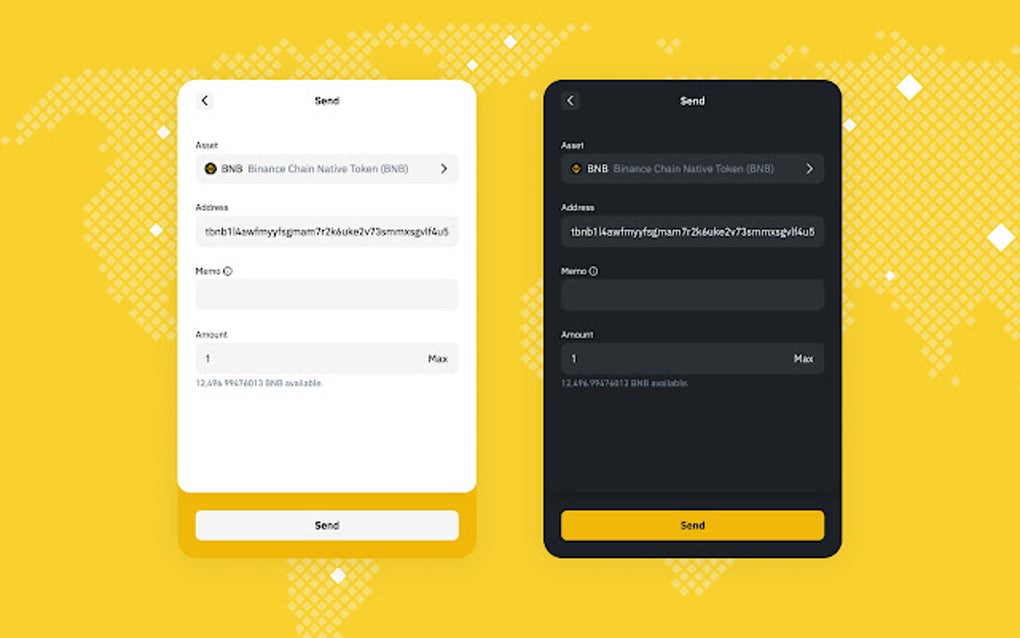The image displays two nearly identical smartphone screens placed side by side, overlaid on a backdrop featuring a yellow world map composed of pale yellow, blocky diamond shapes interspersed with larger white diamonds. 

Both smartphone screens present the same information but differ in color schemes. The displayed data is organized in rows with text boxes. The first row, labeled "Asset," contains the text "BNB Binance Chain Native Token" followed by "(BNB)" and an arrow pointing right. The second row, labeled "Address," includes the text "TBNB1L4AWFRRRGFSGFTAM7R2X6UKE2V73SMMURVH4U5." The third row, labeled "Memo," has a circled 'i' next to it, indicating additional information, and the fourth row, labeled "Amount," shows the text "1MAX." 

At the bottom of each screen is a button labeled "Send." 

The screen on the left features a white background with light gray text boxes and a gray "Send" button, whereas the screen on the right highlights a dark gray, nearly black background, with dark gray text boxes and a yellow "Send" button.